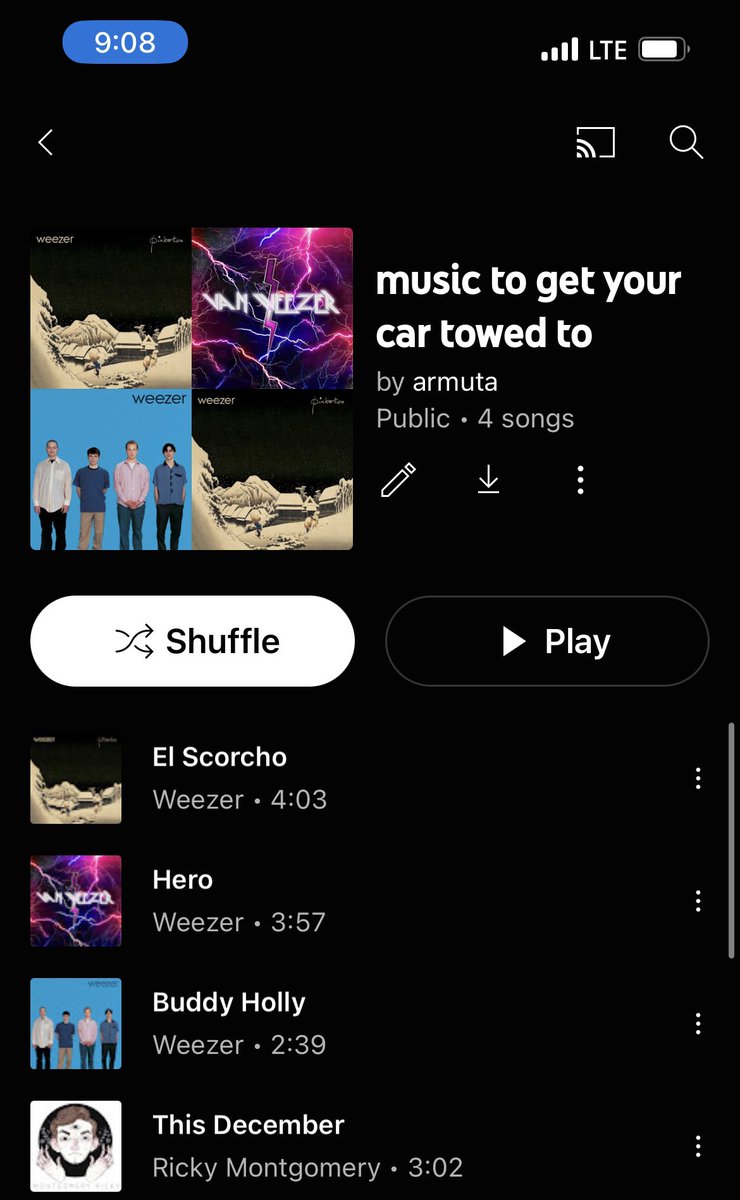This image is a screenshot taken on a mobile device, featuring a mostly black background. The time displayed at the top reads "9:08," written in white font on a blue bubble background. The carrier signal is shown with four bars, indicating strong reception, and the device is connected to an LTE network. The battery icon suggests good battery life. A white arrow pointing to the left is visible at the top left corner, next to a square button with the cast icon and a magnifying glass.

The screenshot captures a music streaming app displaying four albums. Two highlighted albums are by Weezer: one titled "Van Weezer," featuring a lightning-themed cover, and another with a blue background depicting the band members standing and looking directly at the viewer. Adjacent to Weezer's albums, there's a playlist named "Music to Get Your Car Towed To" by Ermuda. The playlist is public and contains four songs. Below the playlist title, there are options for editing and downloading, accompanied by a shuffle button illuminated in white and a play button. The listed tracks include "El Scorcho," "Hero," "Buddy Holly" by Weezer, and "This December" by Ricky Montgomery.